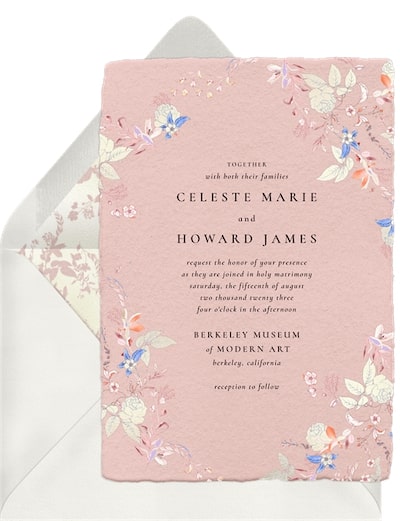This color photograph showcases a wedding invitation gracefully placed atop its accompanying white envelope. The envelope's interior features elegant pink floral embellishments. The invitation itself is crafted from pink, frayed-edge paper, reminiscent of handmade quality, and is adorned with a vibrant floral border featuring white, blue, and orange flowers. Centered on the invitation, in black text, are the words: "Together with both their families, Celeste Marie and Howard James request the honor of your presence as they are joined in holy matrimony. Saturday, the 15th of August, 2023, 4 o'clock in the afternoon, at the Berkeley Museum of Modern Art in Berkeley, California. Reception to follow."